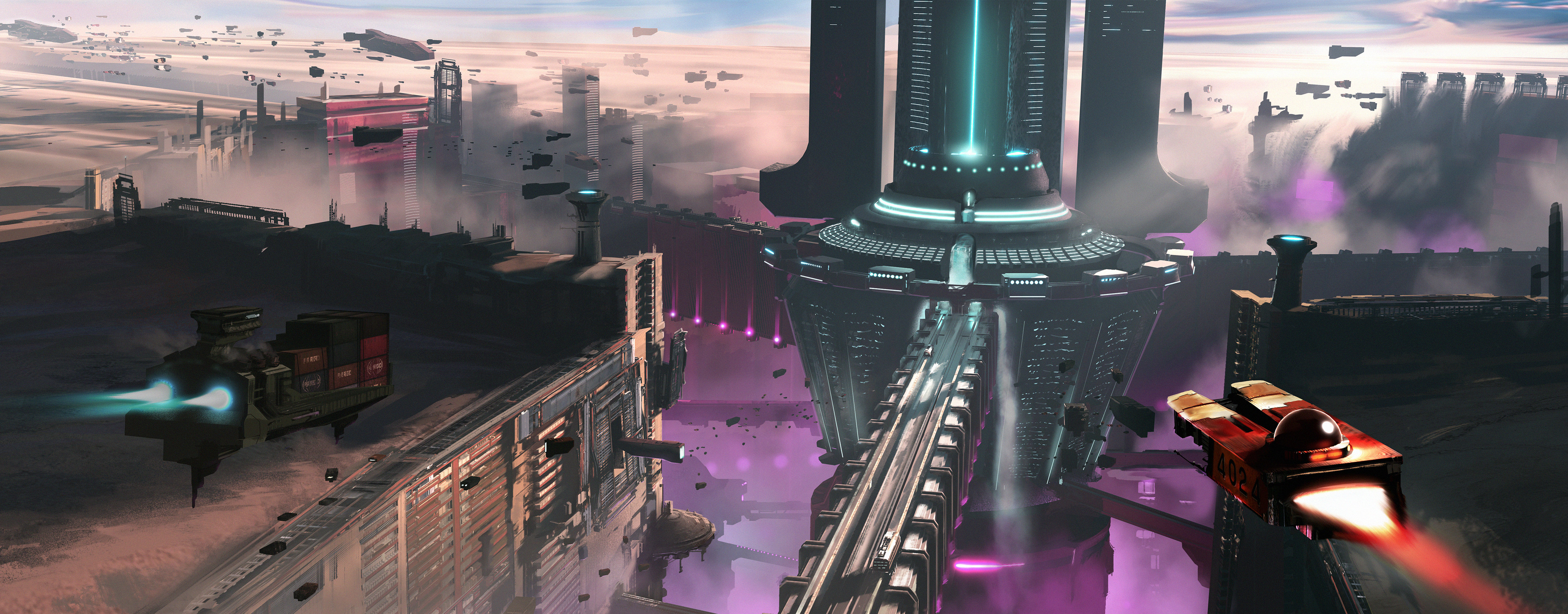The image depicts a highly detailed, computer-generated futuristic cityscape, potentially from a video game. Central to the scene is a large space station or a city floating in the sky, characterized by a prominent, cylindrical structure resembling an upside-down cone with a tall cylinder rising from it, emitting a striking blue laser light. Surrounding this central building are various others, including what appear to be houses on the right and larger city buildings on the left. 

The sky teems with diverse spacecraft, distinct in design and color. On the right, a craft emits a red exhaust fume, while a blue-exhausted craft appears on the left, their unique shapes lacking conventional wings. One rust-colored vehicle has a dome light in front, and another resembles a train, albeit flying as there are no tracks. Beneath the flying vehicles and amidst the futuristic buildings, a possible rail system extends towards the central cylindrical structure. Heavy clouds frame the scene, enhancing the impression that the entire setting is suspended in the sky.